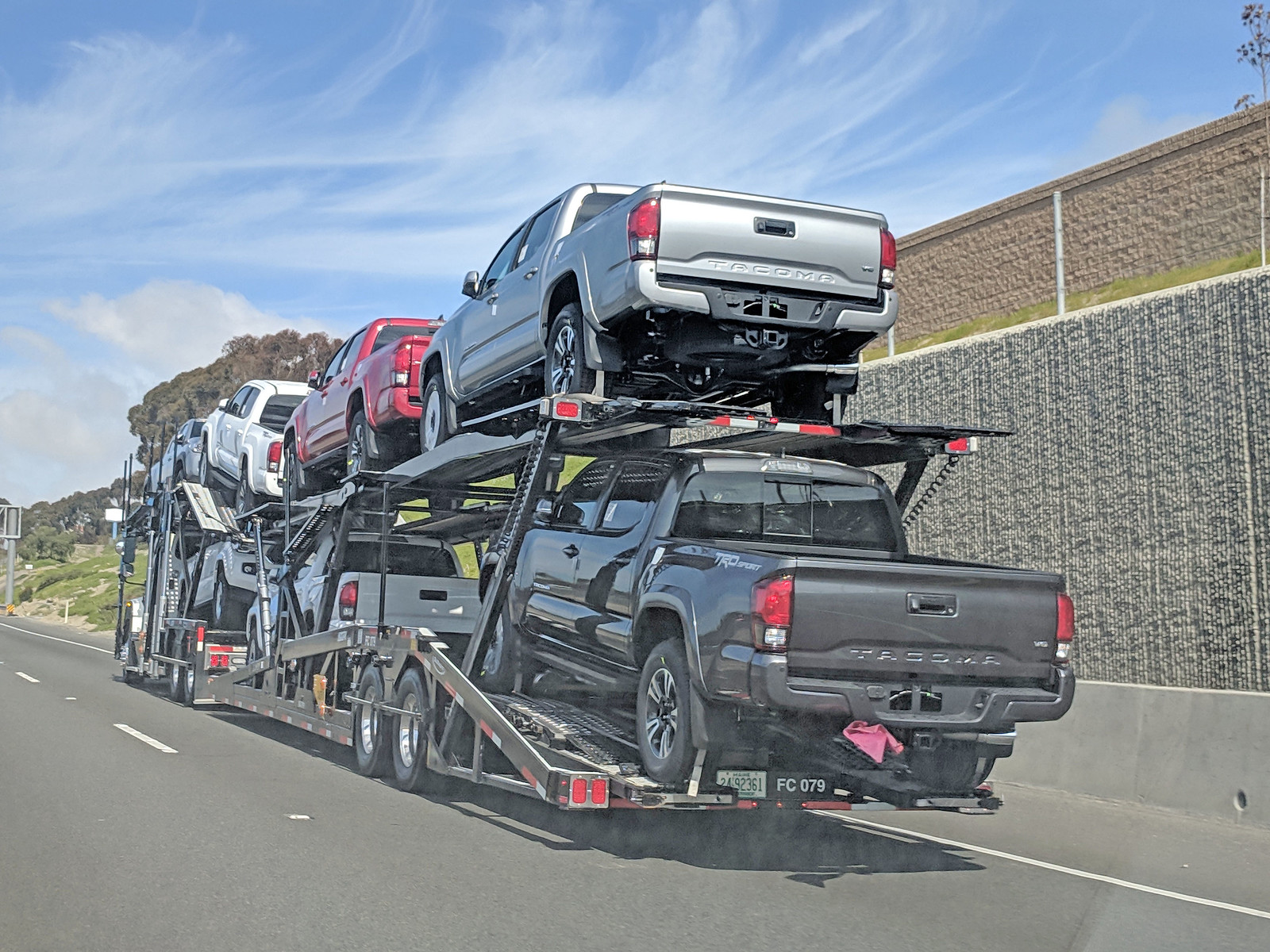This is a detailed photograph of a large transport truck on the highway, likely taken by someone driving in the adjacent lane. The truck is hauling a two-level flatbed trailer loaded with at least eight brand-new Toyota Tacoma pickup trucks. The colors of these vehicles include black, silver, white, and red, with a black one visibly positioned at the back and a silver one above it. The foremost Tacoma appears to be a higher-end Pro Sport model. The truck is traveling in the farthest right lane, passing a concrete retaining wall and surrounded by green, leafy trees. The sky is a clear blue, enhancing the scene's brightness. The back end of the truck displays the identifier "FC 079." Overall, the photograph captures a vibrant and detailed scene of a heavily loaded big rig navigating the highway under a pristine sky.